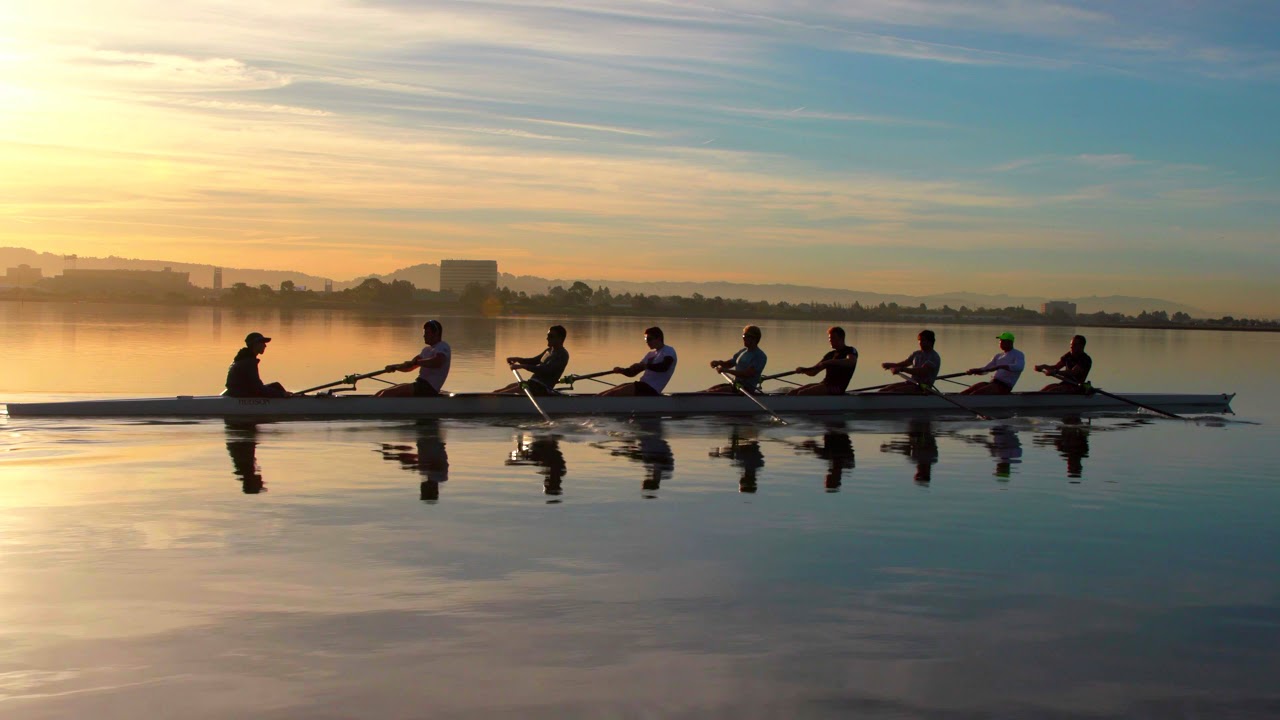In this picturesque outdoor scene, a competitive rowing team of eight men expertly maneuvers a long, narrow rowboat on a calm river. The team members face left, synchronizing their strokes with a single oar each, alternating sides along the boat. At the front, a ninth member, likely the coxswain in a baseball cap, faces them, guiding their pace and commands. The serene early morning or late evening light casts a golden hue over the scene, with the sun just above the horizon in the upper left corner of the image. The sky is a mix of blue hues with wispy white clouds, and the water mirrors this tranquility. A distant shoreline, stretching across the background, adds to the serene beauty of the scene, making it a snapshot of perfect harmony and dedication.